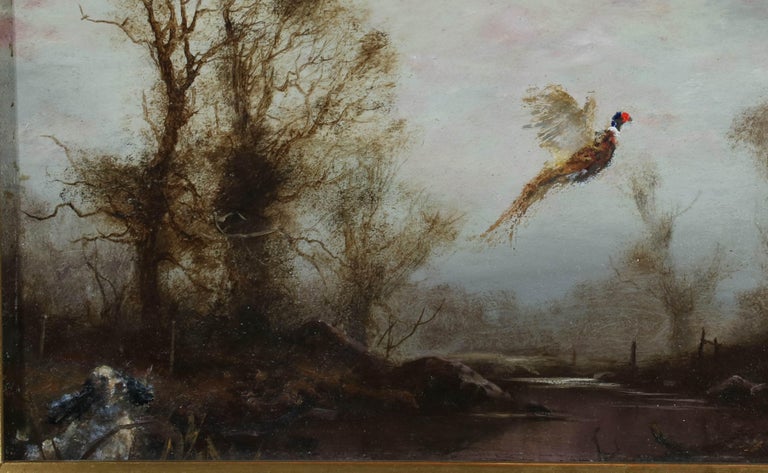This image is an oil painting framed in wood, depicting an outdoor scene set against a somber, gray sky. In the mid-ground, a series of short, wispy trees without green branches stand, leading into a background of more trees. In the left foreground, a large tree stands prominently. The landscape features a slightly hilled terrain beneath these trees, coupled with a small waterway along which several fence posts are visible. Above this waterway, a striking bird with a blue head, red face, and distinctive beak takes flight, wings spread upwards and long tail feathers trailing. In the foreground, a black and white dog with alert, pointed ears is captured looking upwards at the bird. The overall palette of the painting uses darker tones with shades of pastel greys, pinks, blues, and browns, emphasizing the depth and serenity of this valley scene.